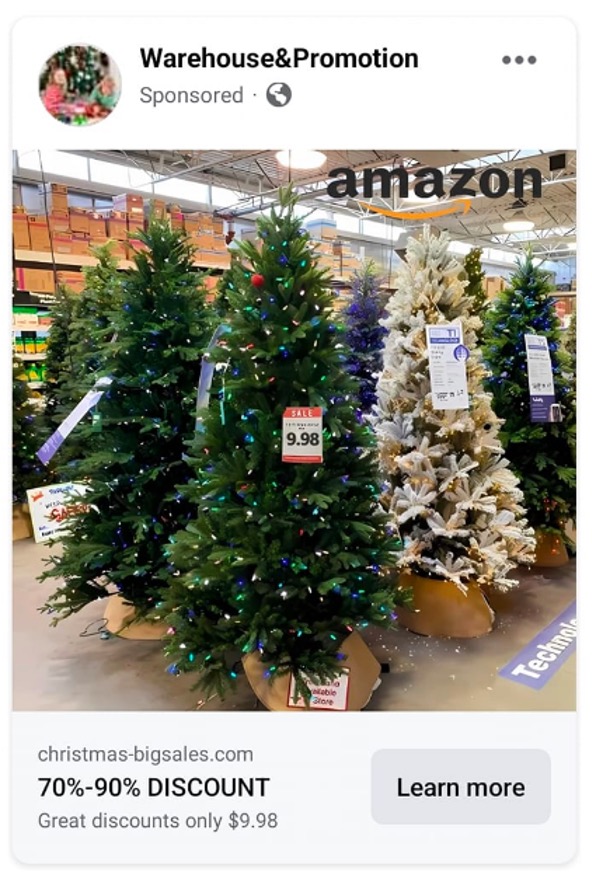The social media advertisement image showcases a promotional post for Christmas trees. The centerpiece is a small, vibrant green Christmas tree adorned with colorful lights in shades of green, blue, purple, and red, standing on a beige, round, hoof-shaped podium. Positioned in the middle of the tree is a sales sign bordered by two red horizontal bars at the top and bottom. The sign prominently displays the price "$9.98" in bold black font. 

To the right of this tree (from the viewer's perspective), there's a similarly sized white and gold Christmas tree, also on a beige podium and decorated with the same festive lights, indicating it is likewise for sale. On the left side of the central tree (from the viewer's perspective) stands another tree of the same hue and also illuminated.

Below the array of trees, the ground is paved with gray concrete. A horizontal white bar spans the bottom of the image, featuring a light gray font that reads "Christmas-big-sales.com". Below this, bold black capital letters announce a "70%-90% DISCOUNT." Further beneath this, in the same light gray font, the text highlights "Great discounts only $9.98 USD", with a grey rounded corner rectangular box to the right containing the words "Learn More" in black font.

In the upper right-hand corner of the image, "amazon" is written in all lowercase black font, and beneath the letters "a" to "n" is a yellow arrow pointing towards the bottom right corner of the text.